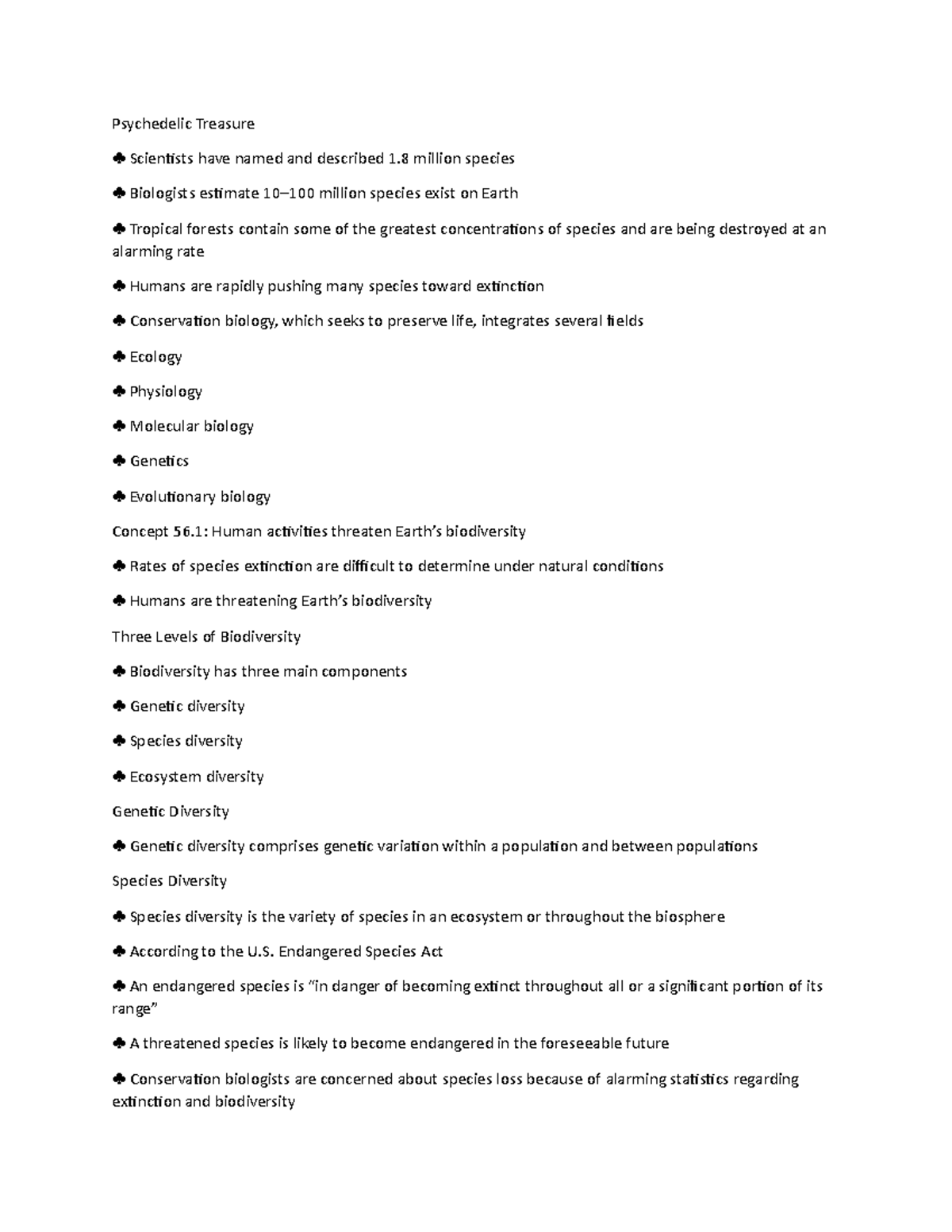**Detailed Caption:**

The image portrays a meticulously structured list set against a pristine white background. Each item on the list is preceded by a spade icon, creating a visually consistent and organized layout. The list is titled "Psychedelic Treasure."

The content delves into various scientific revelations and concerns, beginning with the fact that scientists have named and described approximately 1.8 million species to date. However, biologists estimate that the actual number of species existing on Earth ranges between 10 to 100 million.

A significant focus is placed on the biodiversity housed within tropical forests, which are described as containing some of the highest concentrations of species. Unfortunately, these forests are being destroyed at an alarming rate, contributing to the rapid endangerment and extinction of numerous species due to human activities.

The list further elaborates on ecological and biological disciplines, encompassing topics such as ecology, physiology, molecular biology, genetics, and evolutionary biology. It cites Concept 56.1, which highlights that human activities are a major threat to Earth's biodiversity. It notes the difficulty in determining natural rates of species extinction and underscores the ongoing threat posed by humans to biodiversity.

Biodiversity is discussed across three fundamental levels: genetic diversity, species diversity, and ecosystem diversity. Each of these components is subsequently itemized and detailed, with an emphasis on genetic diversity. The list serves as a comprehensive guide, making complex information accessible through a clear and well-organized presentation.